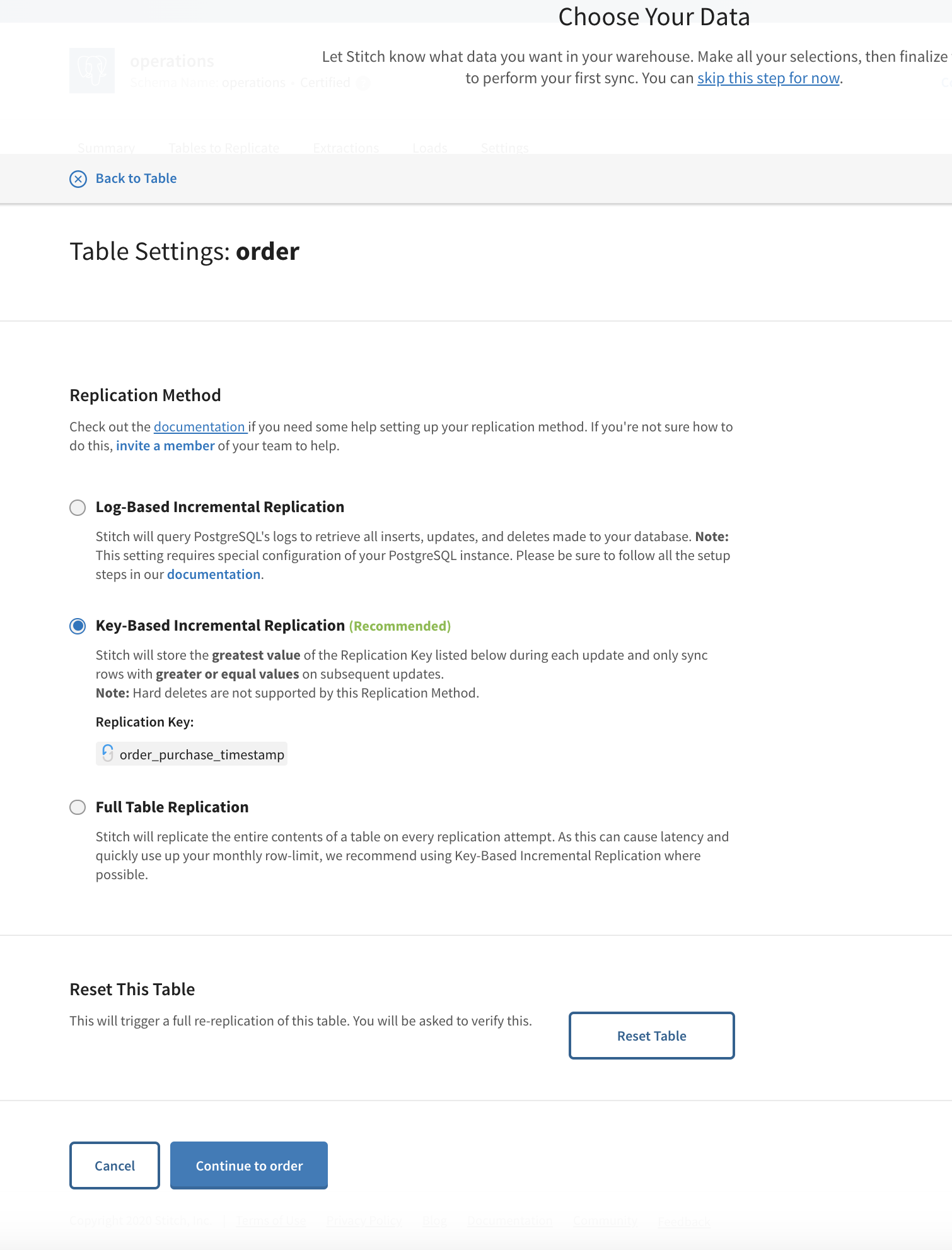The image displays a user interface with the title at the top reading, "Choose your data." Below, it instructs users to "Let Stitch know what data you want in your warehouse." Users are prompted to make their selections and finalize to perform their first sync. A blue hyperlink labeled "Skip this step for now" allows users to bypass this step if desired.

Underneath the hyperlink is a gray box with the text "Back to table." Following this is a section with a white background, headed "Table settings," and it contains the option "Order." Below a light gray horizontal line, the section continues with "Replication method," accompanied by a note to consult the documentation if assistance is needed. It also suggests inviting a team member for help if needed.

The replication methods listed include "Log-based incremental replication," "Key-based incremental replication," and "Full table replication." Each method has a brief description, but the text is too small to read. Each option is accompanied by a clickable circle, with "Key-based incremental replication" already selected.

At the bottom, there is a prompt that reads, "Reset this table. This will trigger a full resynchronization of this table. You will be asked to verify this."